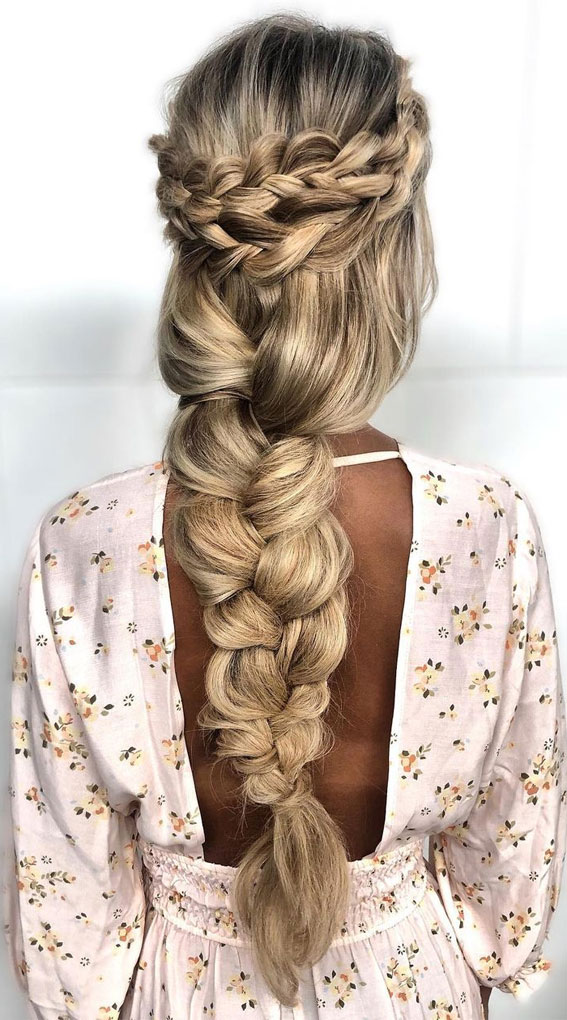This vibrant color photograph captures the back view of a woman with a tan skin tone, standing against a plain white background. She is adorned in a whimsical, long-sleeved, open-back dress featuring a floral pattern of pink fabric scattered with live yellow and orange flowers, reminiscent of polka dots. Her waist-length hair, thicker at the darker roots and transitioning to a lighter blonde, is styled intricately. The hairstyle consists of a loose, twisted braid structured in four layers across the back of her head, blending into a long, cascading braid down her back, intertwined like a Rapunzel-style weave. Additionally, smaller, looser braids wrap around the perimeter of her head, forming a delicate crown or headband.